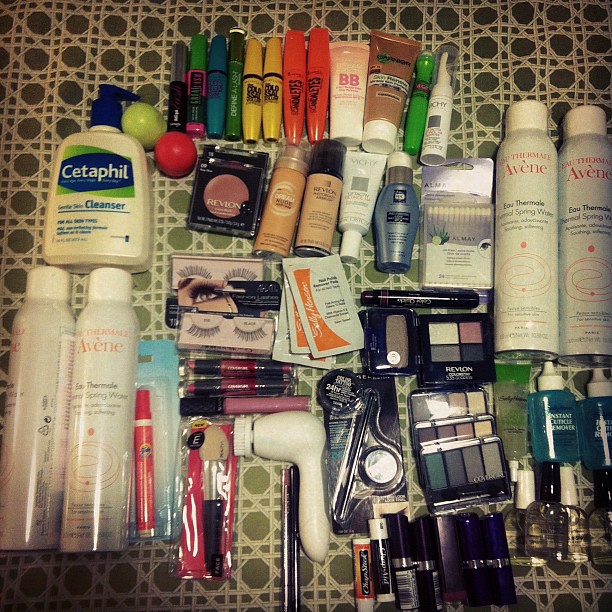The image features an array of makeup, skincare, and body care products meticulously arranged on a green cloth backdrop. The cloth is adorned with intricate white stitching patterns, forming small circular designs where two horizontal stitches intersect with diagonal stitches crisscrossing from the top left to bottom right and vice versa.

Starting from the top left, approximately two inches in, are various-sized cylindrical containers resembling markers in black, pink with a green tip, blue, green, yellow, and orange hues. Directly beside these are two tubes with white caps pointing downward; one is pink, and the other is brown.

To the right of this assortment is a thin green roll-on tube with its applicator visible at the top. Next to it is a white can with a plastic top and an upright nozzle. Following this is a lotion bottle characterized by its blue cap and right-facing pump, completing the upper section.

Amid the layout, a green apple and a red spherical object add a touch of vivid color. Nearby are a bottle of foundation, several elongated bottles and tubes, and a selection of Q-tips and hair products scattered around.

On the bottom row, one can spot more hair products, a Tide stick, a pair of fake eyelashes, a lipstick, a massager, tweezers, and more eye makeup. Notably, there are four eyeshadow palettes—one positioned above and three below. Centered at the bottom are a couple of chapsticks flanked by five lipsticks neatly aligned to the right.

Altogether, the image captures a well-organized collection of beauty and self-care items showcased against a visually engaging patterned fabric.